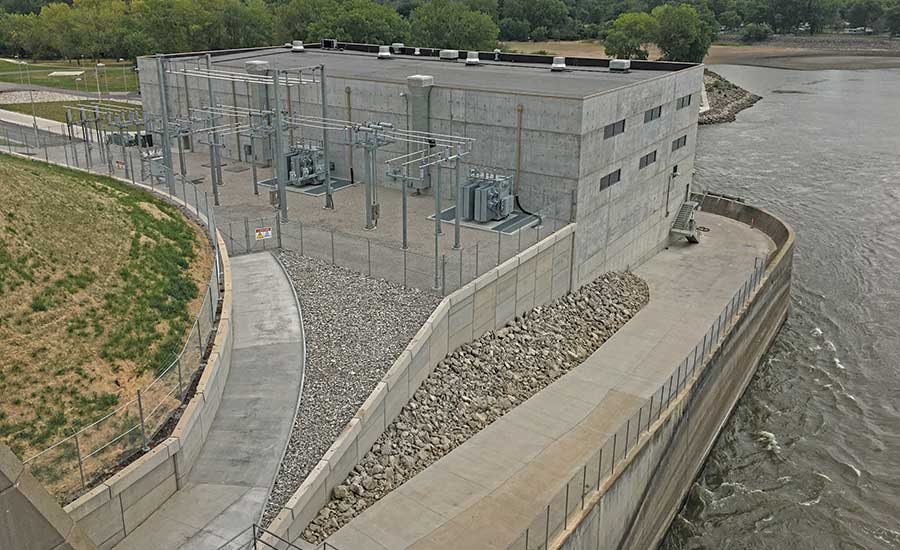The photograph captures a detailed view of a water treatment or power facility situated along a river. The image, taken from an elevated perspective of around two to three stories, shows a concrete building with small, blacked-out windows and various ducts on its rooftop. This building is the focal point, surrounded by an industrial landscape of metal poles and electrical grids, all securely enclosed by chain-link fencing. 

In the right-hand side of the image, flowing water contained by a seawall can be seen extending from the bottom right corner toward the center. This area is bordered by a wide concrete walkway that could serve as a drive, flanked by both gravel and large rocks. In the background, there are sandbars and trees providing a natural contrast to the industrial setting.

On the left side of the building, a ramp leads up to an area with more metal poles, and another sidewalk and fence can be seen in the background. The left side also features patches of scrubby grass and more green lawns that appear to be struggling, with patches of both vibrant and dead grass. Overall, the image depicts the complex infrastructure of a power or water treatment plant integrated into a natural riverside environment, revealing both the industrial machinery and the surrounding landscape.